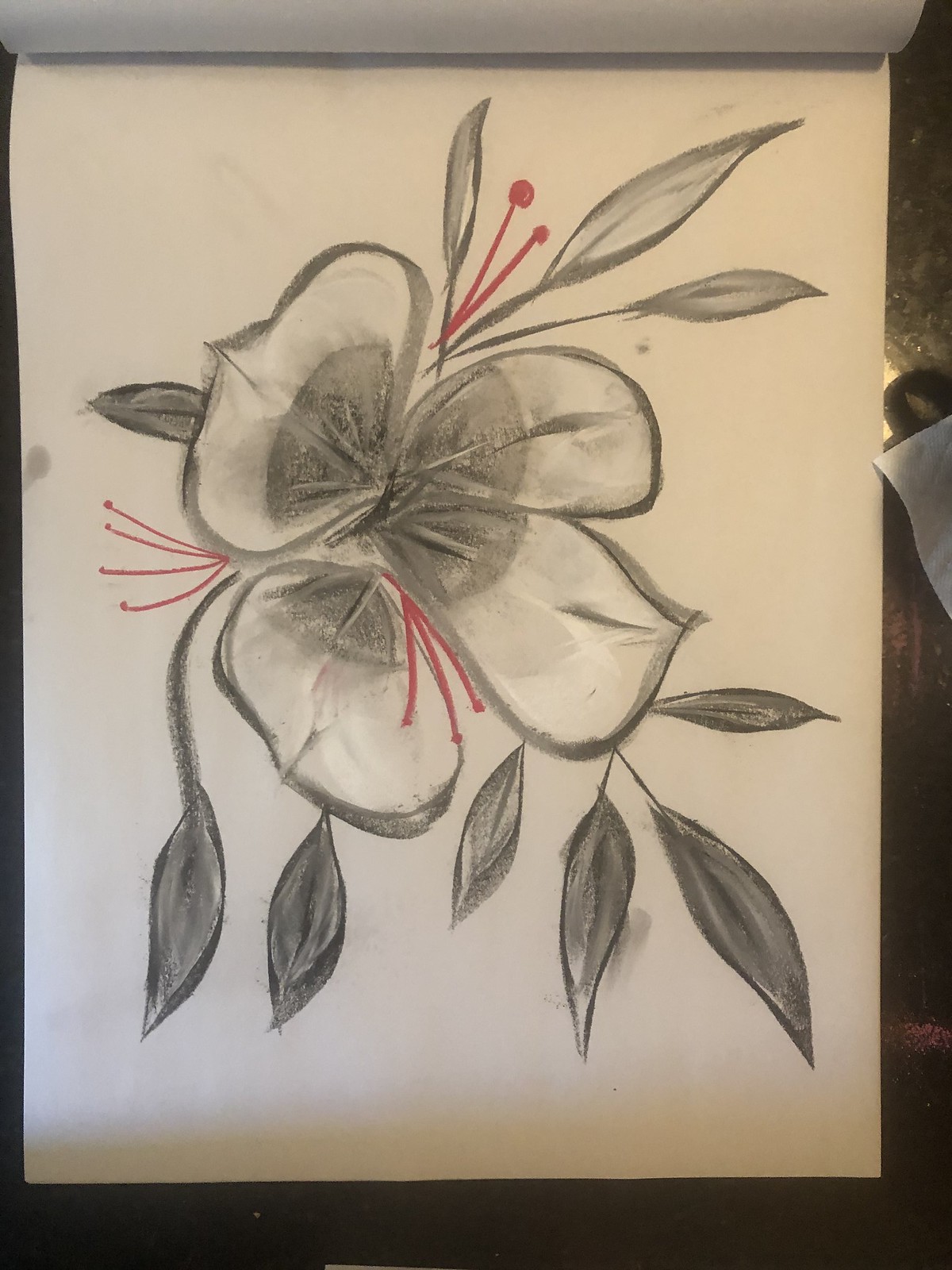This charcoal drawing depicts a single, very large flower rendered on white paper. The flower has four distinct petals, each predominantly white with gray outlining, and the gray color subtly fades into the center of each petal. Encircling the flower are approximately ten narrow, pointed leaves, meticulously drawn with detailed textures. Bright red stamens, which add a striking contrast to the otherwise monochromatic theme, surround the flower, enhancing its visual appeal. This intricate and elegant composition highlights the artist's skill in using charcoal to create depth and contrast.